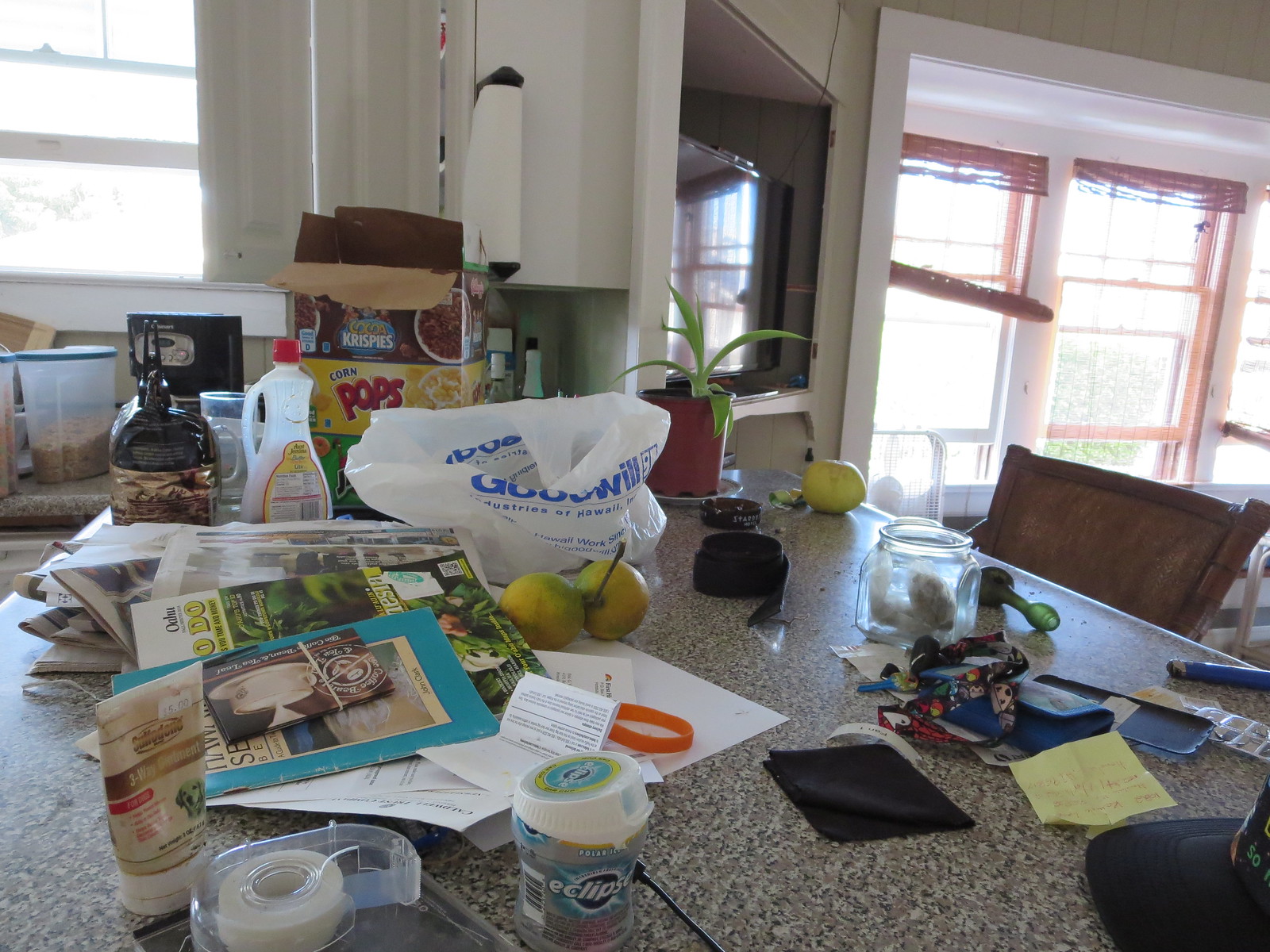### Detailed Descriptive Caption

The image showcases a cluttered kitchen in disarray. Dominating the scene is a large, raised granite countertop, possibly a part of a breakfast bar, suggested by the presence of a bar stool nearby. The countertop is strewn with various items, contributing to its chaotic appearance. Scattered across it are newspapers, both opened and unopened mail, and an assortment of objects including a substantial plastic container of gum, hand cream, scotch tape, and a glass jar holding two or three indiscernible items. There's also an unusual green item with a ball at one end, an onion, a belt, an aloe plant, an almost empty bottle of syrup, a box of Corn Pops cereal, a box of Krispy cereal, and a shiny brown object near the edge of the counter.

Beyond the messy countertop, the kitchen reveals more haphazard elements: Rubbermaid containers filled with dry goods are visible, cabinets stand ajar, and a paper towel dispenser is seen. Extending into the adjacent family room, the scene continues to depict disorder. Pink-colored blinds are half rolled up in a sloppy manner, hanging loose. A fan sits on the floor, and a sizeable TV reflects the windows from across the room. The overall ambiance is one of clutter and unkemptness, capturing a lived-in but untidy space.